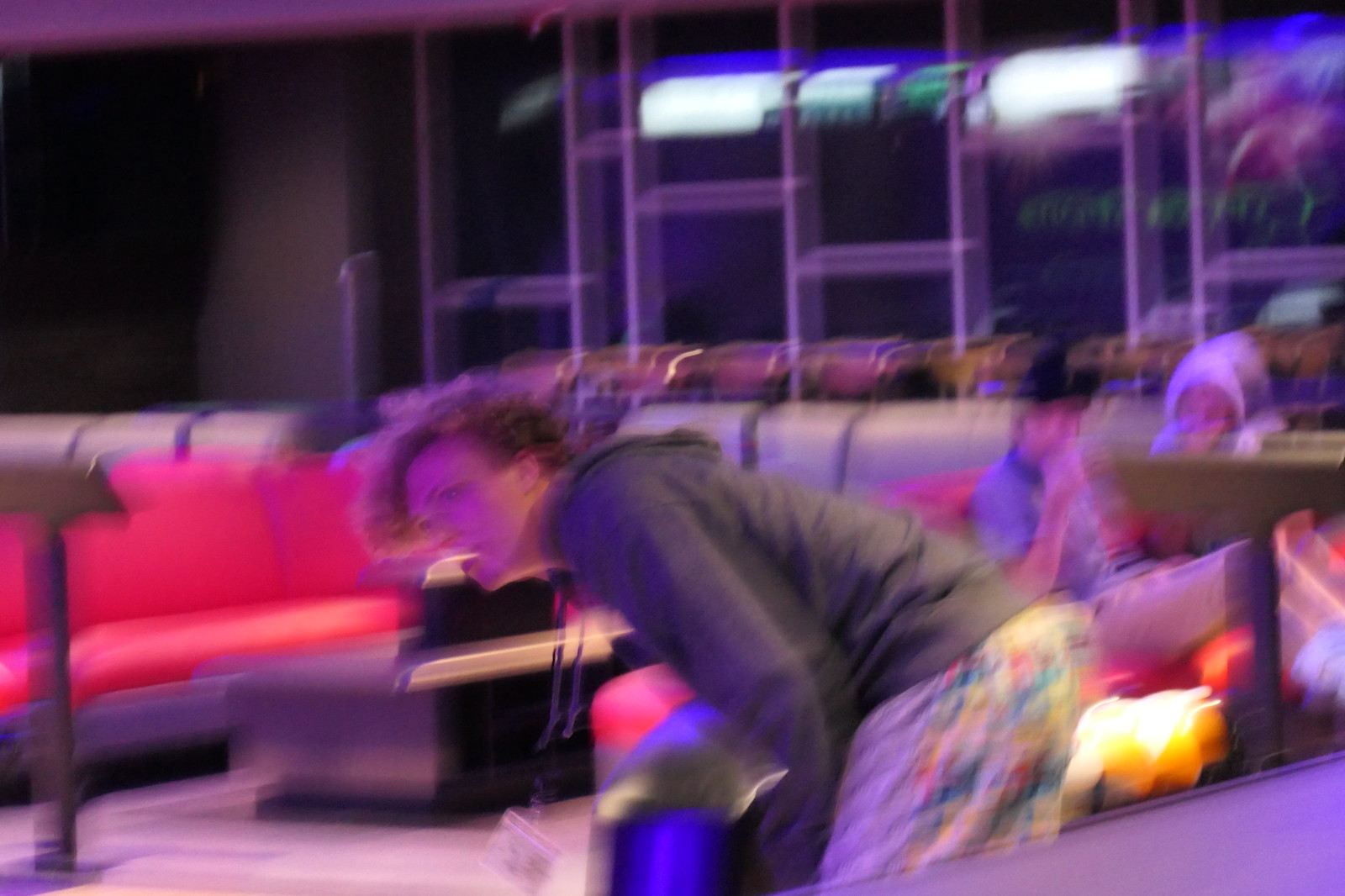In this image, a person is bent over, facing towards the left, captured in a very out-of-focus side view from the right. The setting appears to be a bowling alley. The individual is positioned in front of the ball chute, with the scoreboard area visible at the bottom right—a pole with a flat surface. Towards the bottom of the image, several bowling balls are aligned vertically on a ball return machine. The background features various booths; on the left, they are red, while on the right and farther back, they appear gray. Behind the individual, to the right, more red booths can be seen. Two people are seated in these booths: one man in a blue shirt, black hat, and tan shorts, and another person in a gray hoodie. The top right of the image reveals a wall of windows bordered with metal, while the top left shows a partial view of a gray wall in the background.